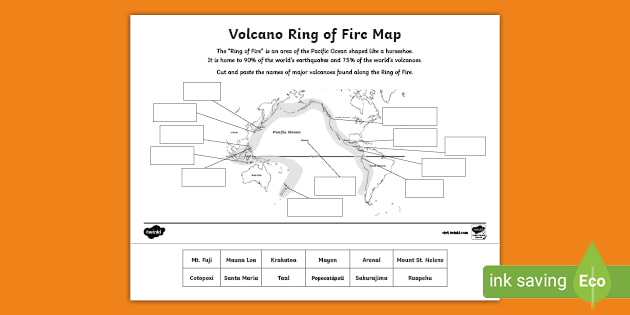The image features a detailed diagram titled "Volcano Ring of Fire Map" at the top, set against a rusty orange background. The diagram itself has a white backdrop with black text and displays the Pacific Ocean surrounded by landmasses including Australia, Russia, South America, and the West Coast of the Americas, illustrating the horseshoe-shaped "Ring of Fire" area. This region is noted for housing 90% of the world's earthquakes and 75% of the world's volcanoes. Below the title, there are six labeled squares with names of various major volcanoes found within the Ring of Fire, corresponding to their locations on the map. Additionally, the bottom right corner features a small green banner with a white leaf graphic and the text "Ink Saving Eco". Text around the diagram provides further context, though some of it is very small and hard to read.